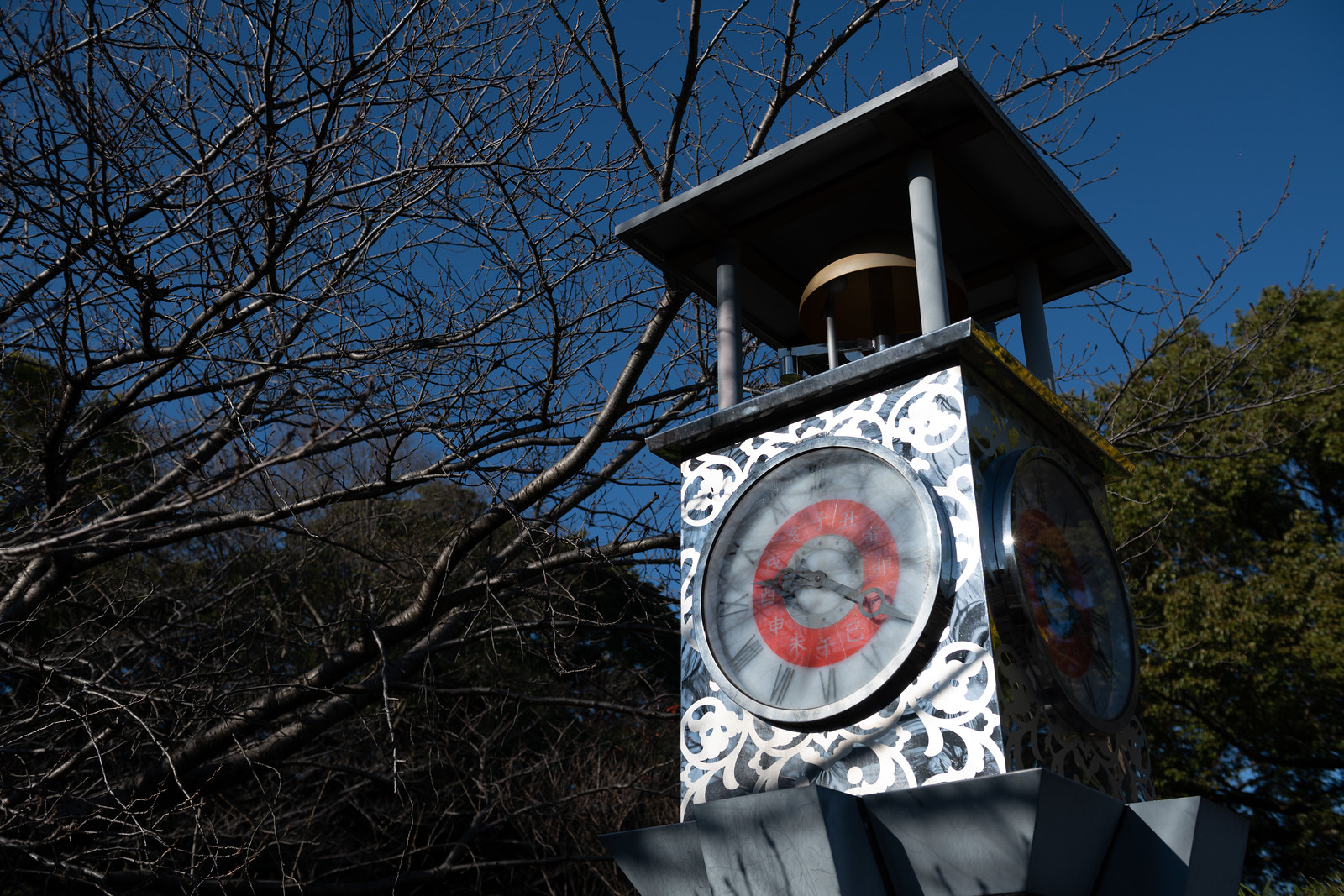The photo captures the upper section of a gray clock tower adorned with intricate, ornamental ironwork in a white lattice design. Dominating the center is a clock face encircled by a prominent silver bezel. The clock itself features Roman numerals and a red ring with Chinese characters around the center, from which the hour and minute hands extend. Above the clock, a large bell sits protected under a cover, likely to shield it from rain. The background contrasts with a vibrant, dark blue sky and a mix of lush evergreen trees and bare, leafless branches, indicating a possible autumn setting. The scene is serene, with the tower standing tall amidst the diverse foliage.